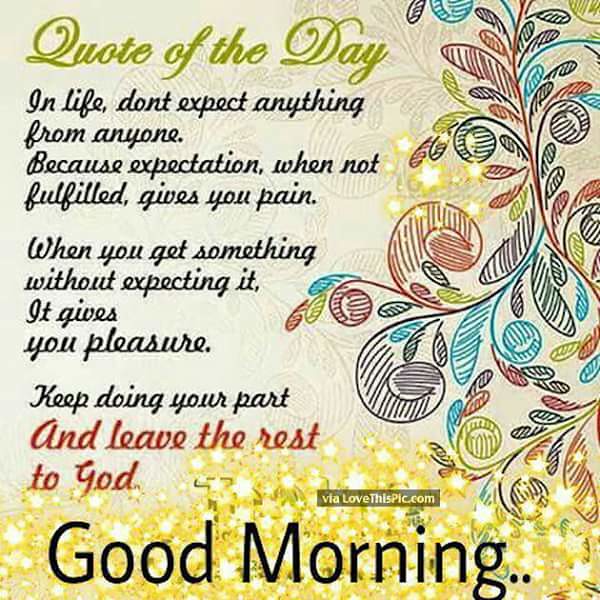The image features a digitally synthesized illustration with a light brown, creamish background adorned with whimsical floral designs. To the right, vibrant, hand-drawn vines and leaves in shades of blue, red, orange, and green stand out against a subtler, darker cream pattern. The bottom of the image sparkles with an array of shiny or yellow stars, resembling Christmas lights. Over these stars, large black text reads "Good Morning." At the top left, in green cursive, the phrase "Quote of the Day" is seen. Beneath it, in black cursive text, is the inspirational quote: "In life, don't expect anything from anyone because expectation, when not fulfilled, gives you pain. When you get something without expecting it, it gives you pleasure. Keep doing your part," followed by the red cursive text, "and leave the rest to God." A small banner above the "Good Morning" message credits the image to lovethispic.com.